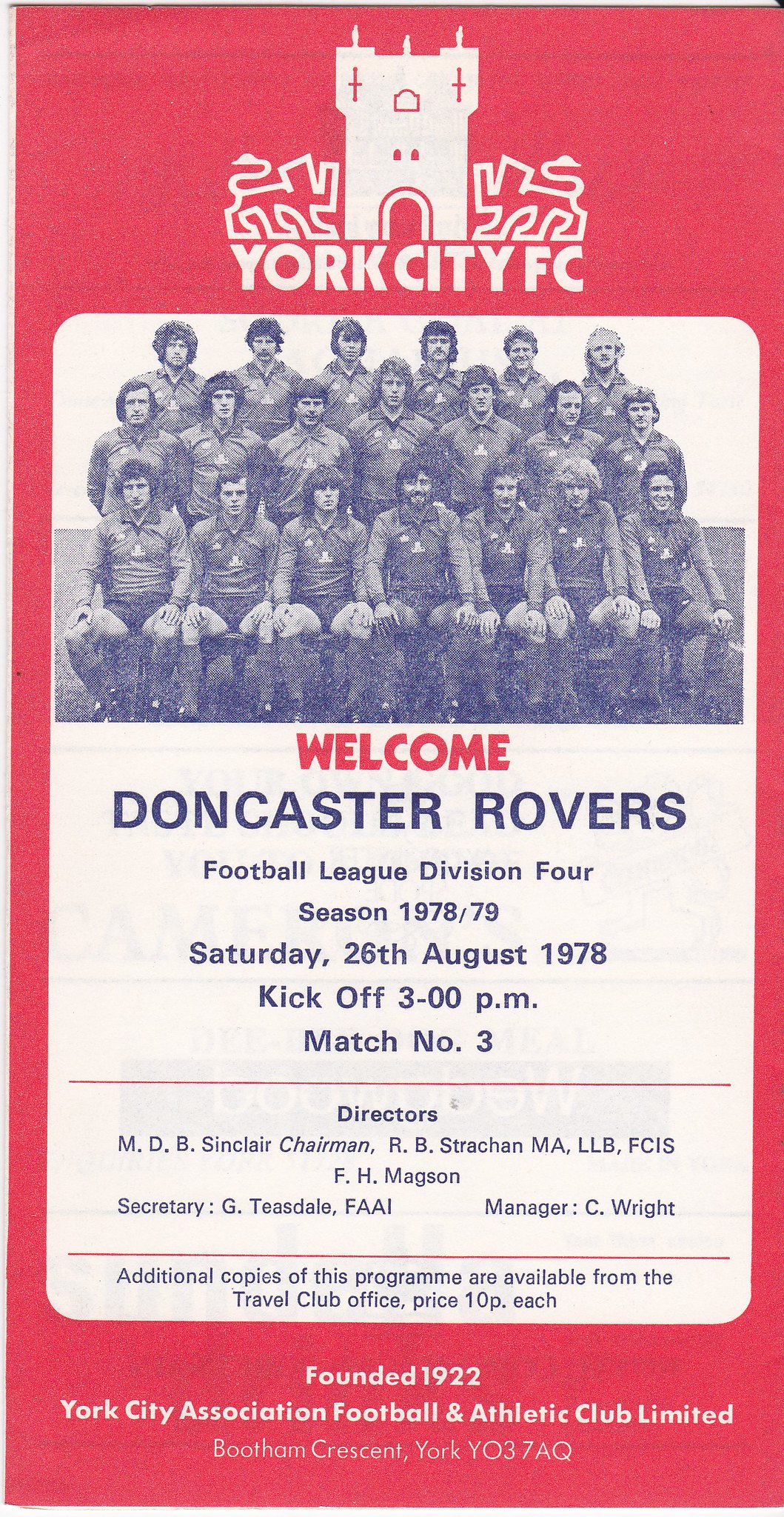The image features the front cover of a vintage sports program booklet, likely from a live soccer game held on Saturday, August 26, 1978, at 3 p.m., match number 3. The cover prominently displays the text "York City FC" alongside a small castle symbol at the top, indicating the soccer club. Below this, there is a photograph of 20 players dressed in their team uniforms, arranged in three rows. The text beneath the photo reads: "Welcome Doncaster Rovers, Football League Division 4, Season 1978-79." Further down, the names of the club directors are listed: M.D.B. Sinclair (Chairman), R.B. Strechin, M.A., L.L.B., F.C.I.S., F.H. Magson (Secretary), G. Tisdell, F.A.A.I., and the manager, C. White. The program, available for 10 pence each from the Travel Club Office, was founded in 1922 as New York City Association Football and Athletic Club Limited. The entire cover is styled realistically with colors including red, white, various shades of gray, dark blue, and black.